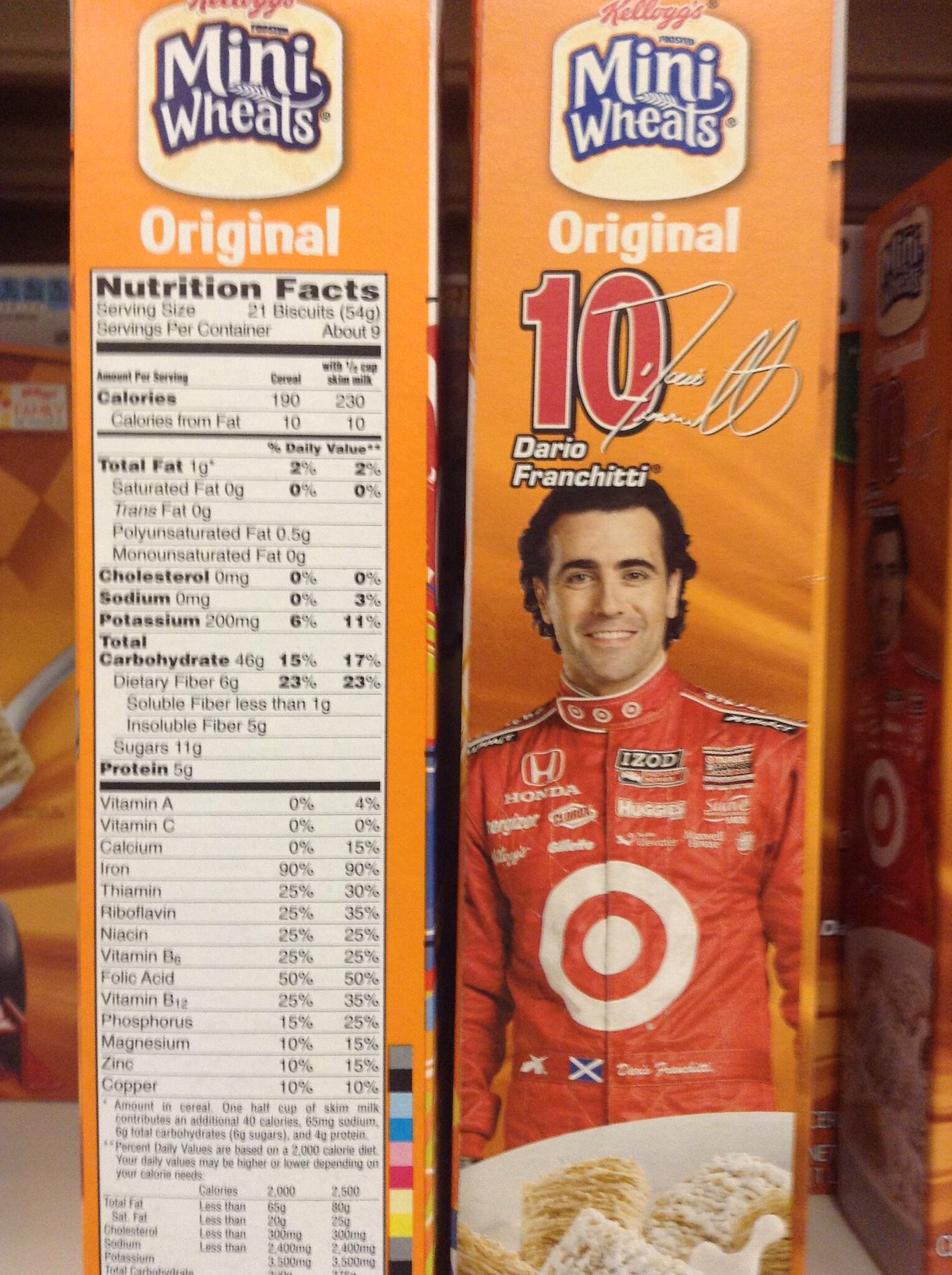This vertically-oriented color photograph captures two boxes of Mini-Wheats cereal placed side by side on a store shelf. The left box prominently displays its black-and-white nutrition facts label, detailing information such as calories, fat content, vitamins, and other nutritional data. The right box showcases a different side, featuring a vibrant image of Dario Franchetti, who is wearing a red jacket adorned with a Target logo and bearing the number 10. At the bottom portion of his box, there is a close-up shot of a bowl of Mini-Wheats cereal. The overall color scheme of the image is dominated by shades of red, orange, and brown. To the right of the boxes, a partial view of another box, likely displaying the same side as the rightmost box, suggests a continuation of the shelf display.